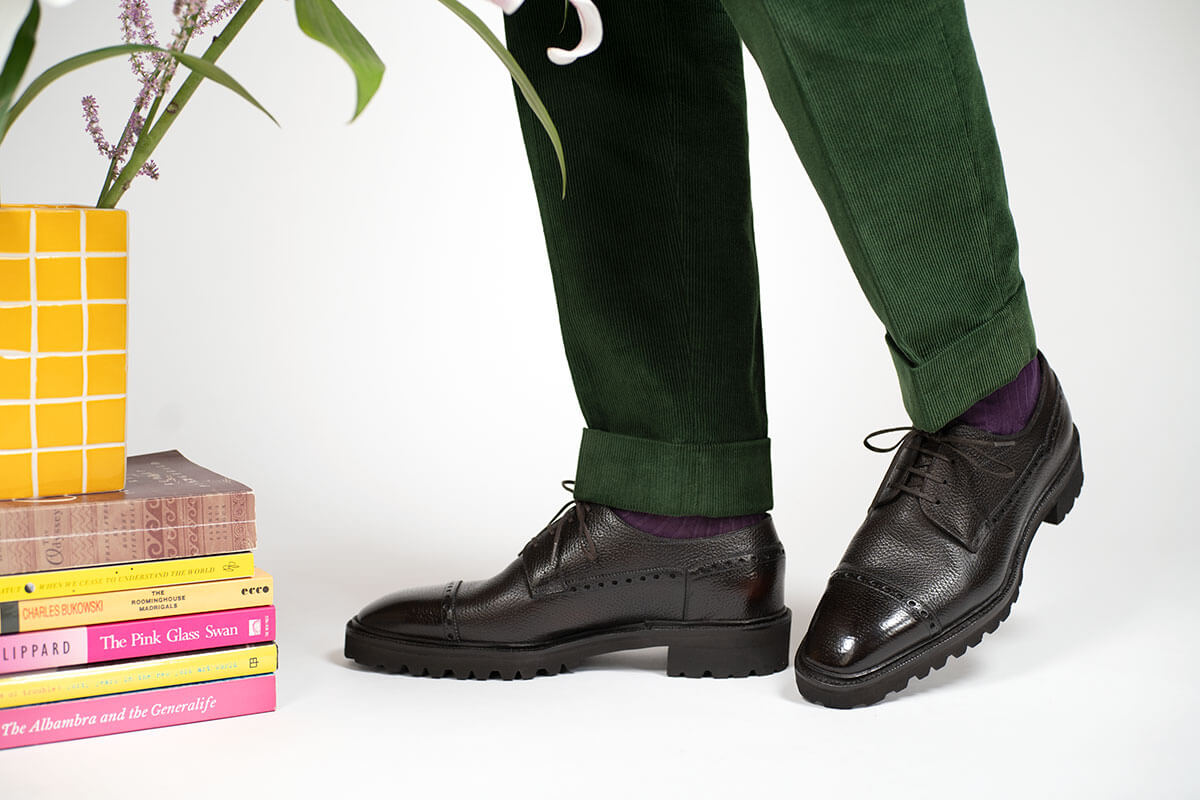In this professionally lit studio photograph with a white background, a person stands with only their legs visible, revealing green corduroy pants cuffed at the bottom, and purple socks. They are wearing polished black leather shoes with thick soles and heels. The right leg faces towards the left side of the image, while the left leg is positioned towards the bottom center. In the lower left corner of the photo, there is a stack of books with colorful bindings: a pink book titled "The Alhambra and The General Life," a yellow book with unreadable letters, and additional books including one titled "The Pink Glass Swan," with other pink and yellow covers. Atop these books sits a white and yellow pot containing a plant with green stems and purple flowers, with a few smaller white flowers scattered around the upper middle portion of the picture.